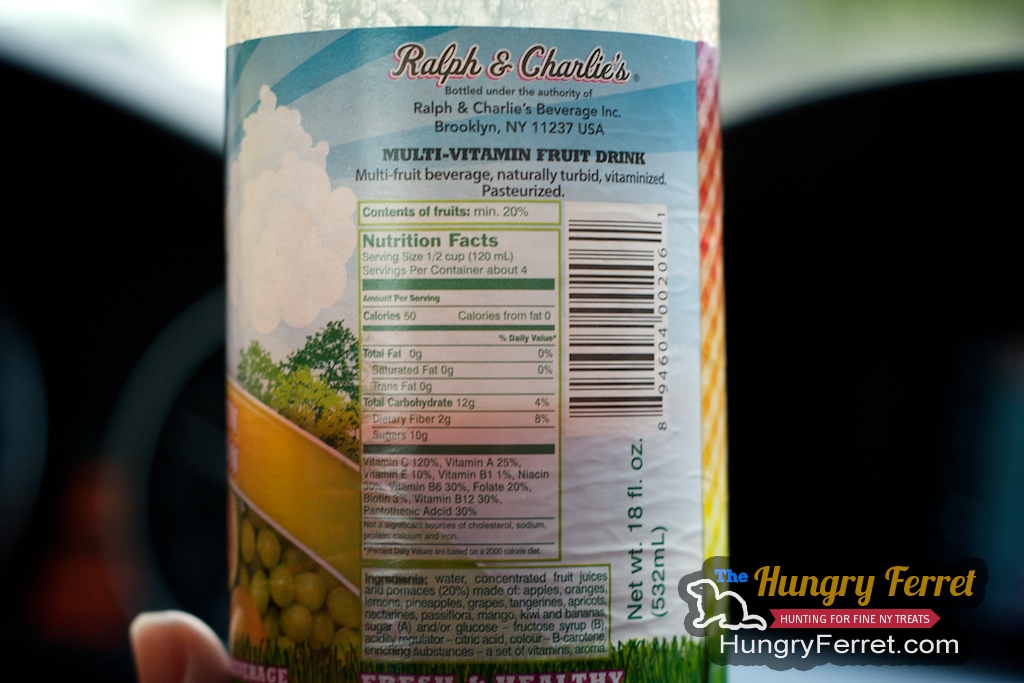This detailed color photograph showcases the back label of a bottle of multivitamin fruit drink. The label prominently features "Ralph and Charlie's" in an elegant script at the top. Below, it states, "Bottled under the authority of Ralph and Charlie's Beverage, Inc., Brooklyn, New York, 11237 USA." The text continues to describe the product as a "multivitamin fruit drink, multi-fruit beverage, naturally turbid, vitamized, pasteurized." Adjacent to these details is your standard nutritional label chart, providing information on the drink’s nutritional content. To the right of the nutritional information, there is a vertical barcode. The image also partially reveals the front of the bottle’s label, where you can see a white cloud, green grapes, and green leaves. Positioned in the lower right-hand corner of the image is the logo of the Hungry Ferret featuring a stylized silhouette of a ferret, accompanied by the website "hungryferret.com."